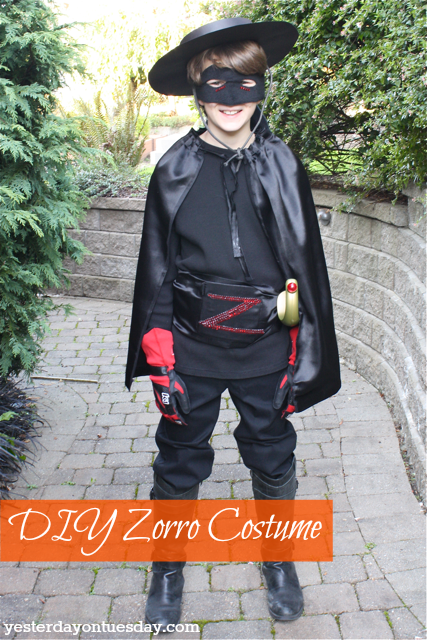The image depicts a young Caucasian boy, likely around 10 or 11 years old, dressed in a detailed DIY Zorro costume. He wears a flat black hat and a black mask that covers his eyes and nose, letting his brown hair peek through. His outfit includes a black satin cape held by a black shirt, a belt emblazoned with a ruby rhinestone "Z," black pants, and knee-high black boots. The boy also dons black and red gloves, holding a gold-handled sword with a single ruby embedded in the hilt. He stands on a stone surface, with a stark gray stone wall and green leaves behind him. Bright outdoor lighting makes the scene clear. The bottom left corner of the image includes text in white letters on an orange background that reads, "DIY Zorro Costume" from "Yesterday on Tuesday.com."